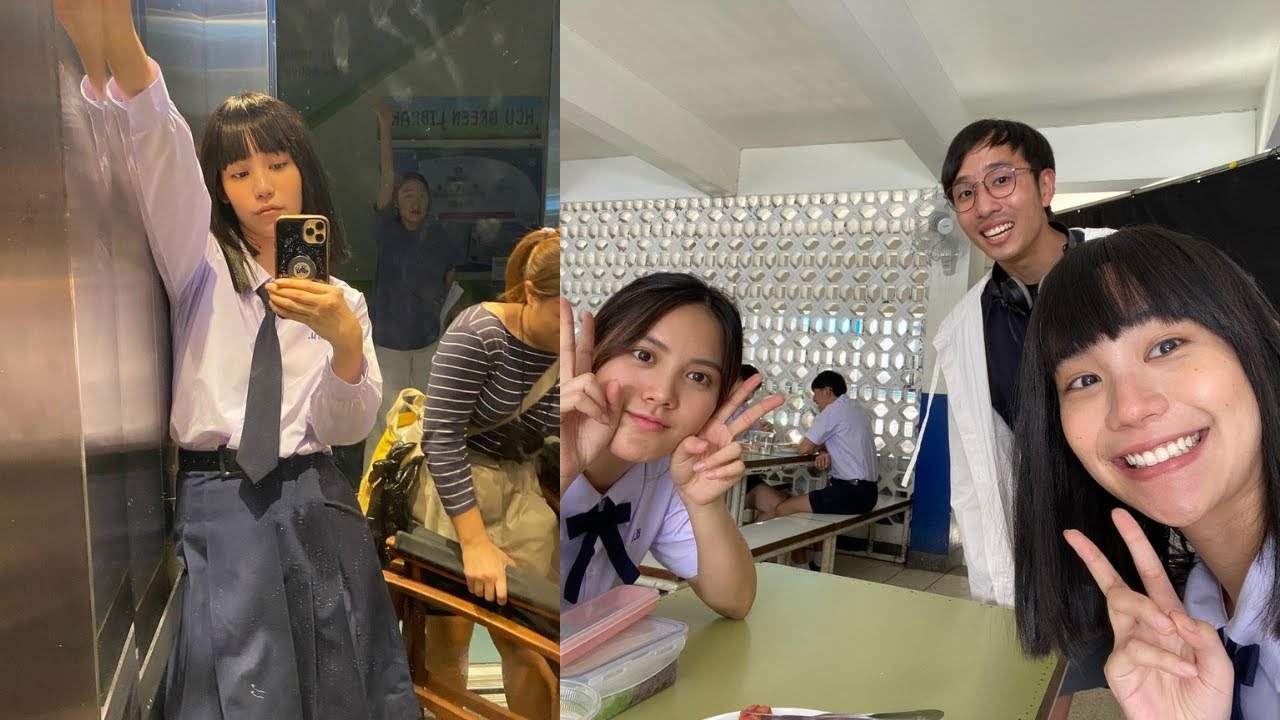The image consists of two side-by-side photographs focusing on young East Asian individuals taking selfies. The left photograph features a young girl with long black hair, dressed in a formal outfit consisting of a white long-sleeve shirt, a gray skirt, and a gray necktie. She is leaning against a mirrored wall with her arm raised and holding an iPhone Pro to capture the selfie. Behind her is a woman dressed in a navy striped shirt and khaki pants, carrying an item, while another girl in the background is partially visible, raising her right arm.

The right photograph shows the same girl with two other individuals. One girl is sitting across from her, flashing peace signs with both hands, while another girl, possibly the same as in the left photo, is standing behind her, making a peace sign with her right hand. Both are smiling at the camera. A young man with glasses stands behind them, also smiling, leaning into the frame. They appear to be in a social setting, possibly a cafeteria, with a picnic table and other students visible in the background against a backdrop that includes a plastic wall divider.